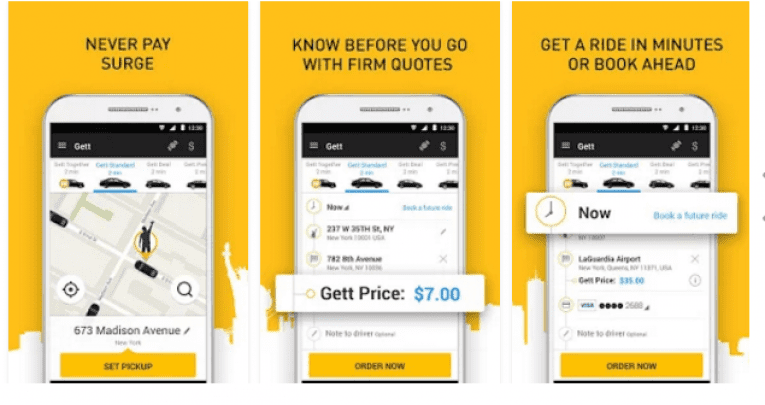This series consists of three photos, aligned side by side, each separated by a white border. These rectangular images, all in portrait orientation, collectively display a cityscape pattern at the bottom, beginning on the left with the Statue of Liberty and continuing seamlessly across the next two images.

Each photo features a yellow background with a black font overlay and showcases a smartphone at its base, suggesting a transportation-related app similar to Uber. Here's the detailed break-down:

**Photo 1**: 
- At the top, the text reads: "Never pay search."
- The phone display shows an image with a black border, a text starting with "Get," and a graphic of several cars, hinting at a ride-sharing service.
- The screen also displays an address: "637 Madison Avenue," and a yellow box labeled "Pickup."

**Photo 2**:
- The header text says: "Know before you go with firm quotes."
- The phone's screen highlights a blue box with the text "GETT $7," indicating a fixed price for a ride.
- Further details suggest the app provides guaranteed quotes.

**Photo 3**:
- The text reads: "Get a ride in minutes or book ahead."
- The phone display shows a clock icon and a yellow box with the text "Now," suggesting immediate service availability.
- Another option states: "Book a future ride," indicating the app allows for ride scheduling with known prices beforehand, promoting efficiency and convenience.

In summary, these photos collectively advertise an app that offers fixed-price transportation services, immediate ride booking, and future scheduling, all wrapped in a user-friendly presentation.